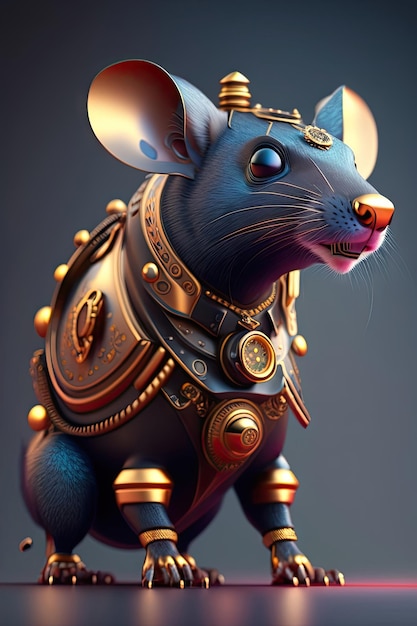In the highly detailed computer-generated illustration, a black mouse is strikingly adorned in elaborate golden armor. The armor, which is meticulously smooth and cleanly rendered, envelops the mouse's torso with protruding, circular plates and extends to golden bands around its front legs. Its claws and feet are similarly armored in gold, emphasizing the protective gear's intricate detailing. The mouse's head features a golden helmet with additional armor pieces centered on top, framing a large, beady brown eye that contrasts against its golden nose and ears. Notably, the armor on its neck includes a collar housing a dial, possibly a compass, and a round shield with an emblem on the side. The setting showcases a blackish-gray background and a gray floor with reflections and a hint of red along the floor line, adding depth and realism to the scene.